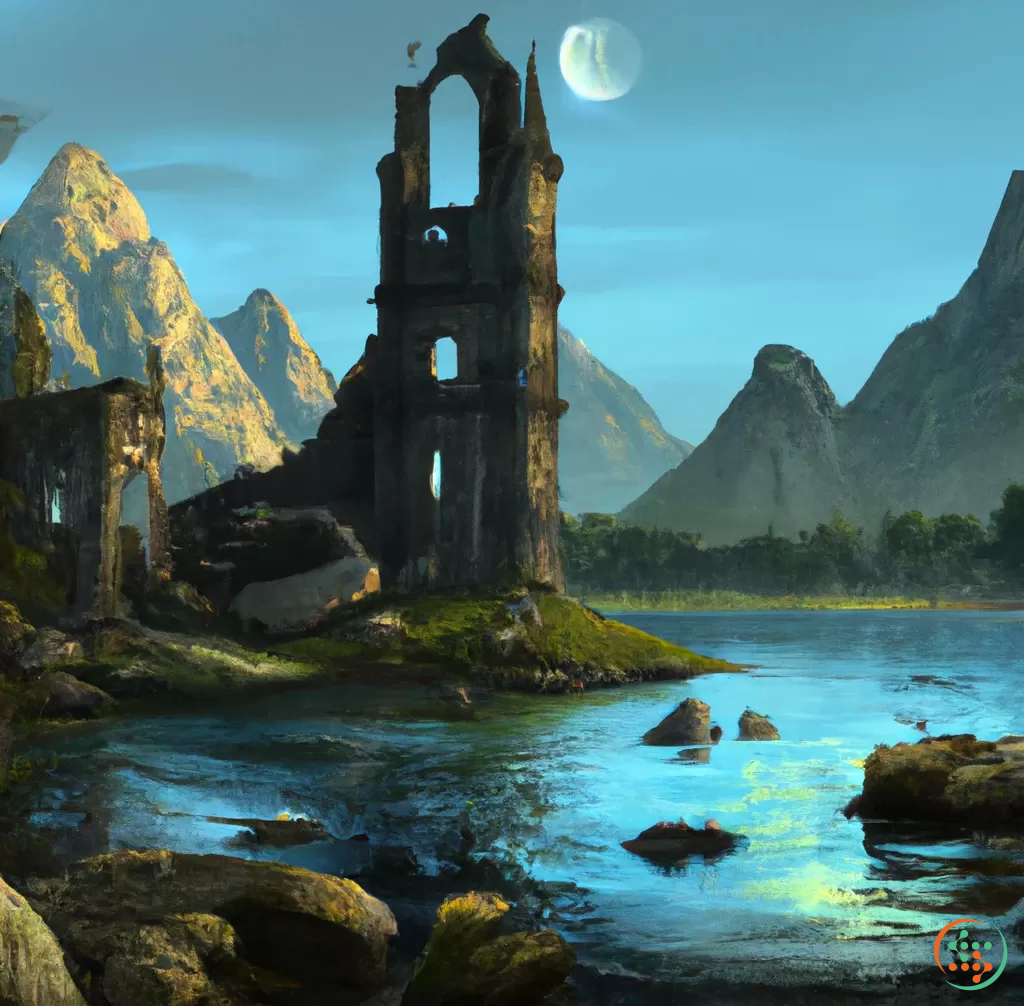This painting portrays a mystical, fantasy landscape at dusk, where the surreal ambiance is enhanced by glowing hues of green and blue. A luminous, cracked moon hangs in the light blue sky with streaks of grayish blue, casting an ethereal light over the scene. Towering, narrow mountains rise dramatically along the horizon, while a dilapidated, once-grand castle stands on a small island in the middle of a lagoon. The castle, reduced now to a single tower, stairs, and an archway entrance, is surrounded by a serene body of water that curves gracefully into the foreground. Scattered large boulders and verdant trees add texture and depth to the tranquil scene, which feels like a hidden refuge, perfect for mythical creatures to dwell.